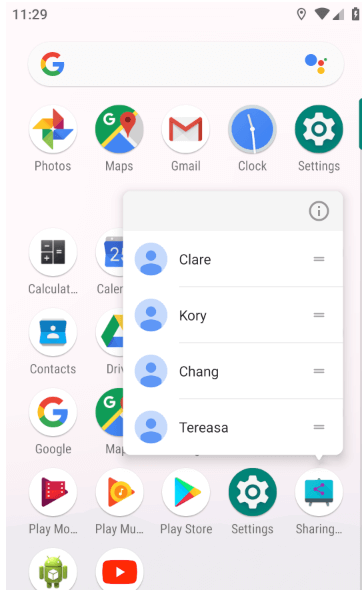The image depicts a smartphone screen with a beige background. At the top of the screen, a row of circular app icons is visible, each accompanied by a label underneath. The apps include Google Search, Photos, Maps, Gmail, Clock, and Settings, among others. In the foreground, a sharing app interface has popped up, displaying a small rectangle listing four friends’ names. Beside each name, there is an icon showing a simple silhouette of a head and shoulders within a circle, indicating user profiles. The names listed are Claire, Cori, Chang, and Teresa, each with a corresponding blue icon. Towards the top left of this rectangle, there is a blank box with a lowercase 'i' enclosed in a gray circle, suggesting additional information is available.